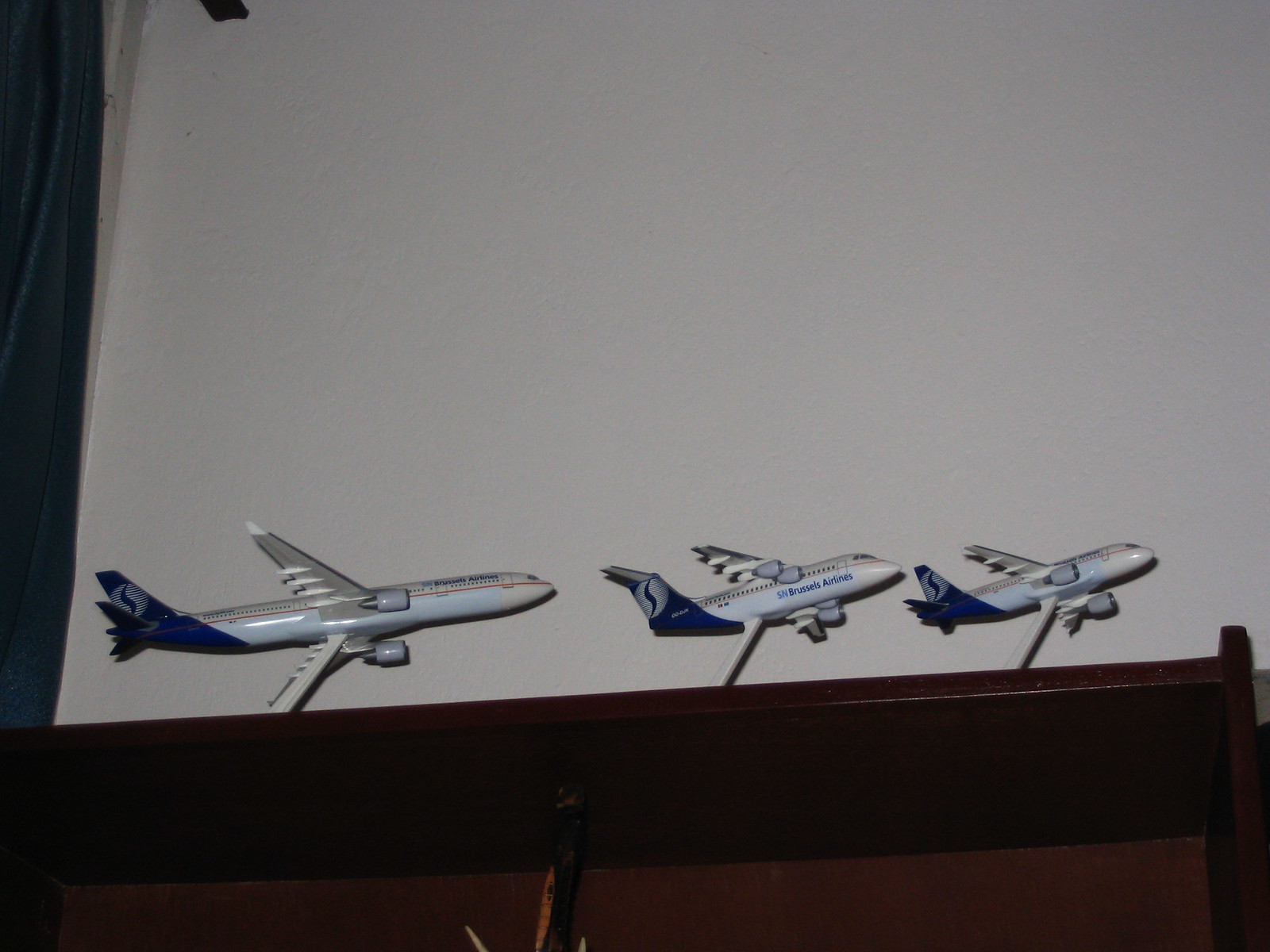The image is a slightly wider-than-tall illustration with a focus that is not exceptionally sharp but adequate to discern the details. Dominating the bottom third of the illustration is a dark brown wooden bookcase or shelf, providing a foundation for the scene. Perched atop this shelf are three model airplanes, varying subtly in design. Each aircraft is primarily white with distinctive navy blue tail fins. The planes rest on small stands, giving the illusion that one wing from each plane touches the shelf while the other points upward. The background is uniformly white, reminiscent of a projector screen or poster board, enhancing the models' prominence. To the far left, a green curtain is partially visible, adding a touch of color to the scene. The planes show variations: the one on the far left resembles a 747, the middle one perhaps a 727, and the rightmost looks like a smaller 747 or potentially a Douglas model. The cohesive arrangement suggests a meticulous graphic design approach, lending a 3D effect to the entire composition.